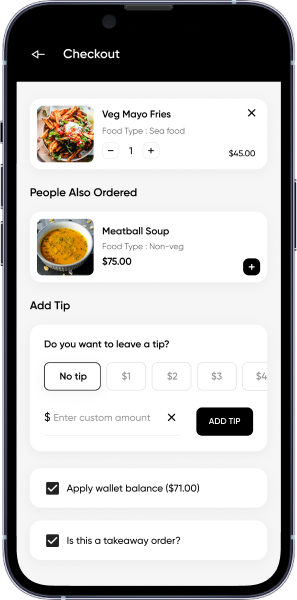This image features a smartphone with black bezels, showcasing a photoshopped screen simulating a food delivery app interface, reminiscent of platforms like Uber Eats. The screen displays a grey background with a prominent white rectangle at the top, detailing an item entry. The highlighted item is "Veg Mayo Fries," written in black font, accompanied by an image of a bowl of fries topped with a scoop of mayonnaise situated to the left. Below the item name, it is categorized under the food type "Seafood." Adjacent to this are buttons for adjusting the quantity, marked with a minus and plus sign centered around the number "1." In the upper-right corner of the item section is a small 'X' icon. The price for the Veg Mayo Fries is indicated as $45, which appears unusually high. Below this, a recommendation section titled "People also ordered" suggests another item: "Meatball Soup." This section includes an image of a bowl of soup, categorized under "Non-veg," and priced at $75.